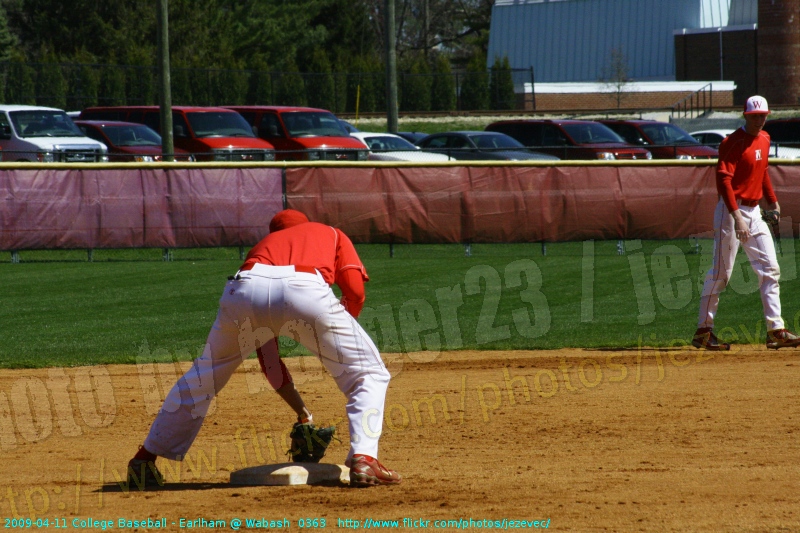The photograph, taken from home plate on a sunny day, captures an intense moment during a baseball game. The scene features two players in matching red long-sleeved jerseys, white pants, and dark shoes. The player closest to the camera, bent over near first base, touches the base with his gloved left hand. To his right stands another player on the boundary between the brown dirt infield and the lush green grass outfield. In the background, a fence, possibly made of burgundy and dark brown plastic fabric, separates the field from a parking lot. This lot is lined with various vehicles including multiple red vans, a white van, a burgundy truck, a white car, and others, against a backdrop of dense green trees and a tall gray metal building. The bottom of the image is marked with text, noting "2009-4-11 College Baseball, Earthlum, at wabash0363," along with a photo credit to "Badger23/jeze."